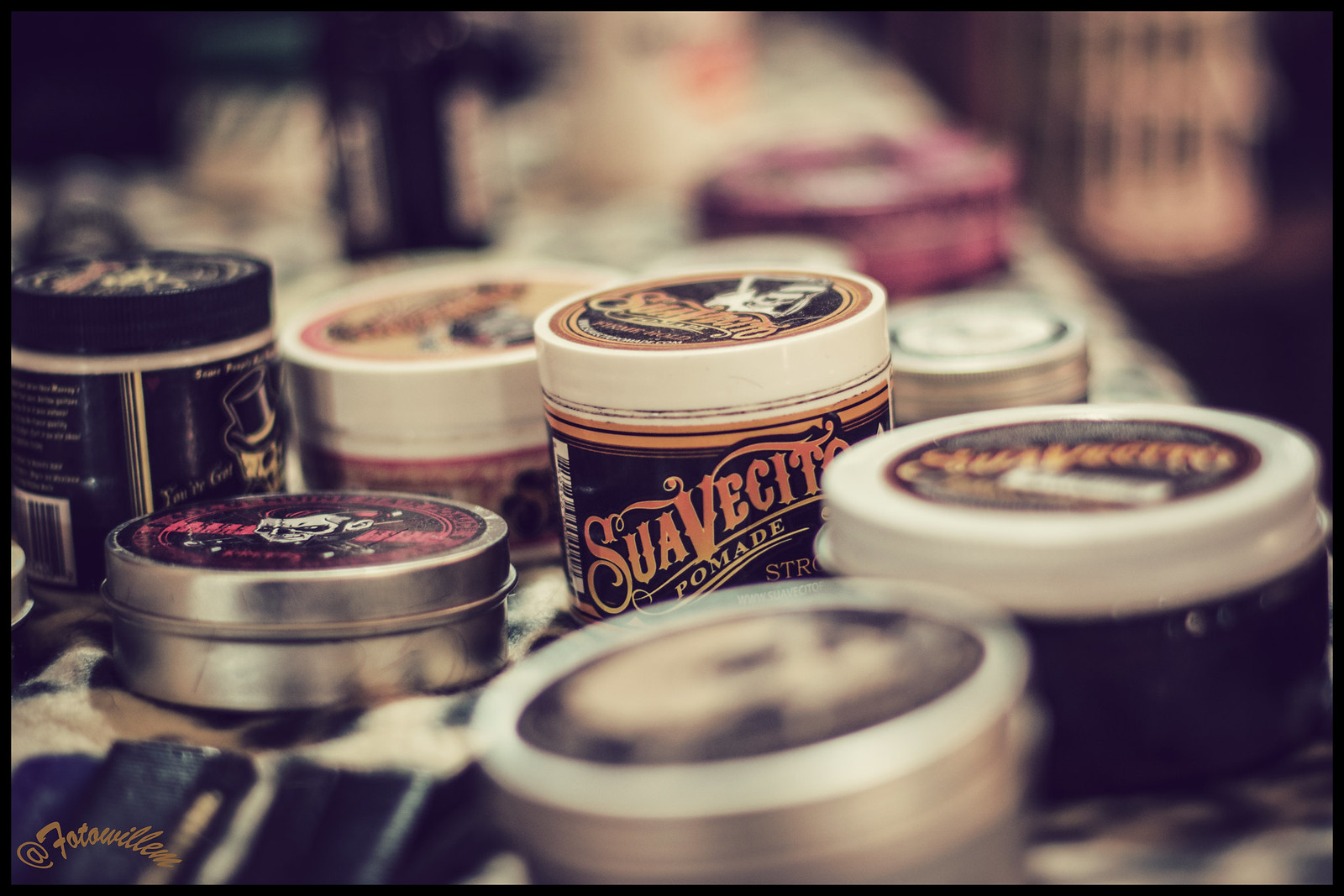The image showcases a variety of small cans and containers arranged on a shelf, prominently featuring hair care products. The containers display a mix of materials, including metal surfaces, and colors, with some featuring a black and white design. The centerpiece is a vertically positioned jar with a distinctive logo in black, bordered by orange lines and adorned with orange letters that taper to yellow at the bottom. The logo prominently reads "Suavecito," with "pomade" in gold beneath it within a border, and the letters "S-T-R" visible underneath. Additionally, there’s another can with a skull illustration and hot pink lettering next to it. The containers appear used and slightly dirty, particularly around the openings. The image has a thin black border, and at the bottom left corner, there's an "@volovillage" handle in yellow. Although many of the cans and features are blurred, the visible details and the mix of vibrant colors contribute to the overall cluttered yet vibrant scene.